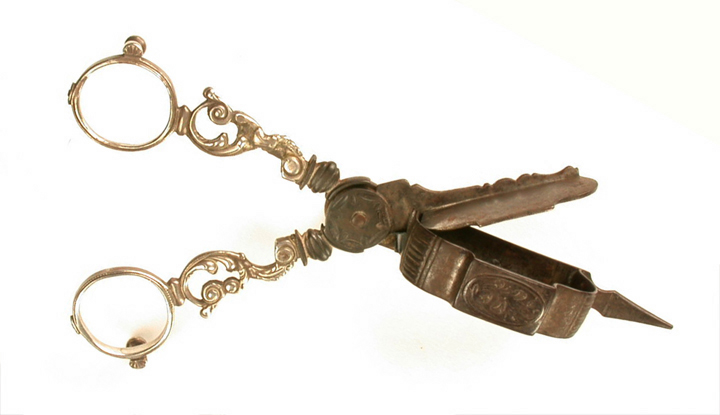This image depicts a highly ornate and antique device resembling a pair of vintage scissors. The handles, designed for the thumb and forefinger, are circular and intricately adorned with gold-toned, steampunk-esque detailing. The design is elaborate, featuring wavy and carved metal work that adds to its decorative appeal. Unlike typical scissors, the functional ends do not have sharp blades; instead, they form a small metal canister with a lid. When the handles are squeezed together, this action closes the lid on the canister, suggesting it may have been used for compressing or containing small objects. The box, which appears to be made of pewter or a similar metal, is equally ornate and features meticulous metalwork. At the very tip of the device, there is a small metal point, adding to its unique and intricate design.